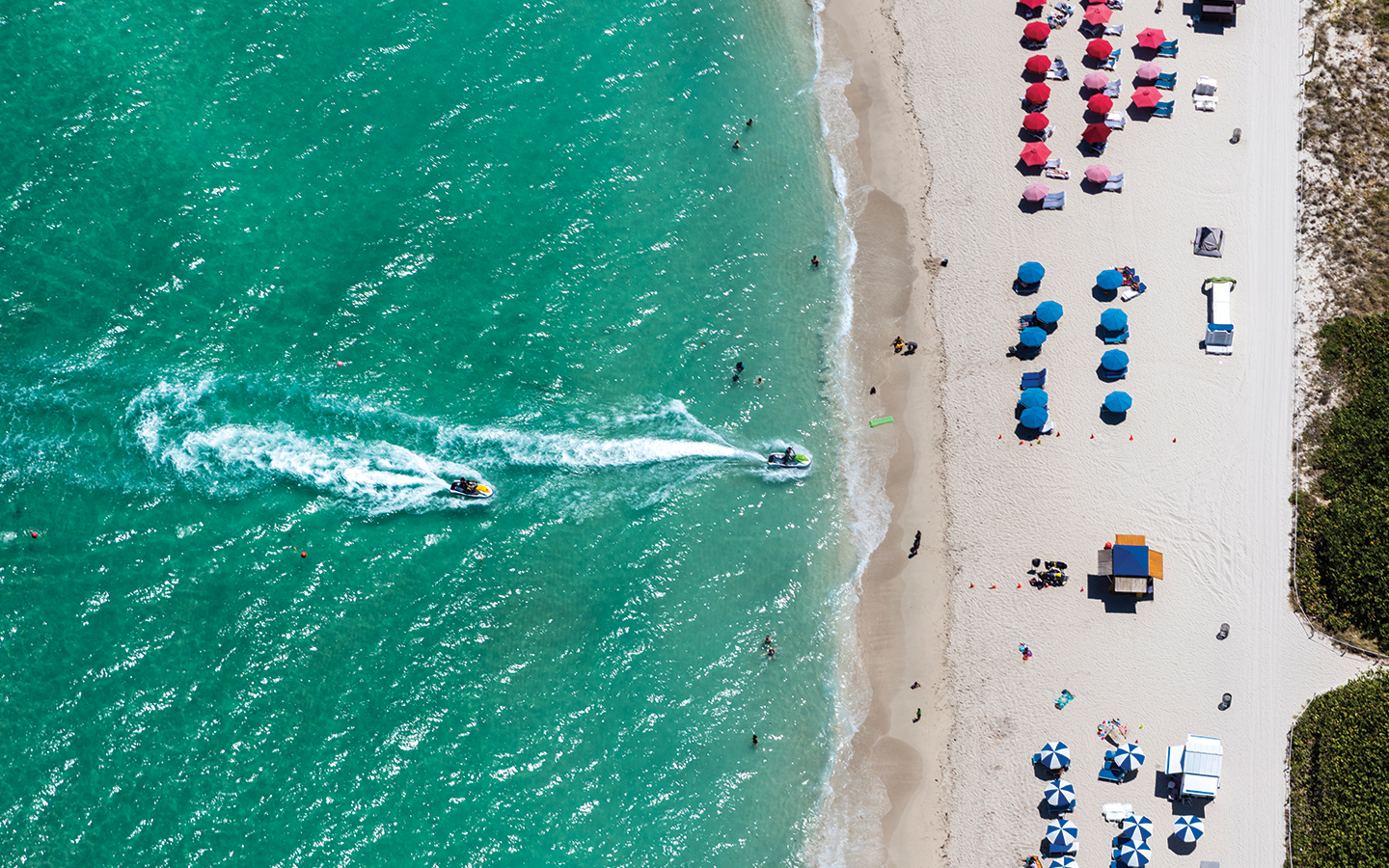This is an aerial photograph, likely taken by a drone, capturing a vibrant beach scene in landscape orientation. The image features a striking contrast between the teal ocean on the left and the white sand beach on the right. Two jet skis create white wakes as they race toward the shore, one closer to the beach and the other slightly farther out. Scattered throughout the water, a few people can be seen swimming.

On the beach itself, there are groups of people walking and a few standing near the water's edge. The main beach area is punctuated by clusters of colorful umbrellas: in the top right section, there are predominantly red and pink umbrellas with lounge chairs underneath; in the center, a cluster of nine blue umbrellas; and at the bottom, a group of blue and white striped umbrellas in front of a blue and white shack, which presumably rents out the umbrellas. Behind these, a small structure with a flat roof and four panels—two gray and two orange—provides additional shade. Bordering the right edge of the beach is a patch of greenery, adding a touch of nature to this idyllic coastal scene.